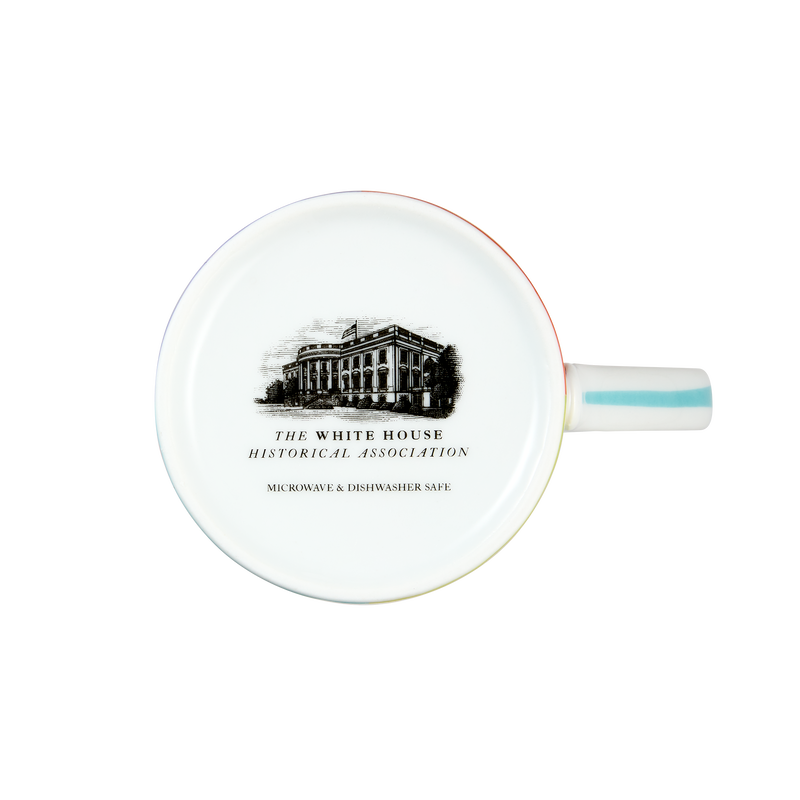This is a photographic image depicting a white china plate with an orange border, set against a completely white background, likely indoors. The plate features a detailed black-and-white line drawing of the White House, complete with a flag on top. Below the illustration, text reads “The White House Historical Association Microwave & Dishwasher Safe.” There's no other text visible in the image. On the right side of the plate, a white handle with a horizontal blue band suggests that it might be the bottom of a mug instead of a plate. The image’s simplicity is emphasized by the lack of any background or additional decorative elements.